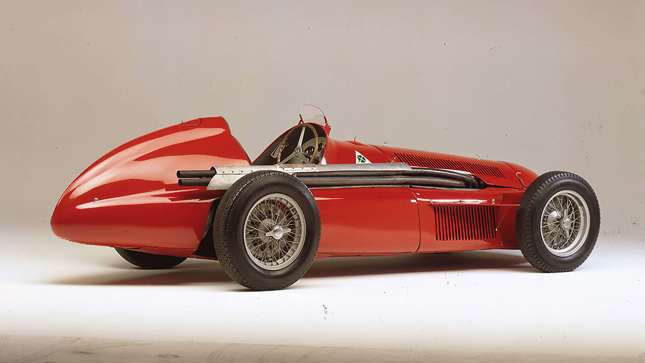The photograph is a full-color, horizontally rectangular image staged indoors with artificial lighting. The background features a gray wall and a white floor, illuminated from the left side. At center stage is a sleek, red, 1960s-style race car. It boasts a long, thin, low-to-the-ground design that is almost as short in height as the wheels themselves.

The race car is a one-seater, having only a cockpit without traditional seats or doors, indicating that the driver must climb in from the top. The cockpit is located towards the back, where the car's body curves, and a small windshield, or visor, extends just to eye level above a standard, round steering wheel.

With black tires and fancy rims, the car is a study in compact performance. Its shiny red body is complemented by an exposed silver exhaust pipe that starts at the front under the hood, running along the side above the back wheel. The car is parked immaculately on the white floor, casting a distinct shadow, indicating the careful control of artificial light in this indoor setting.